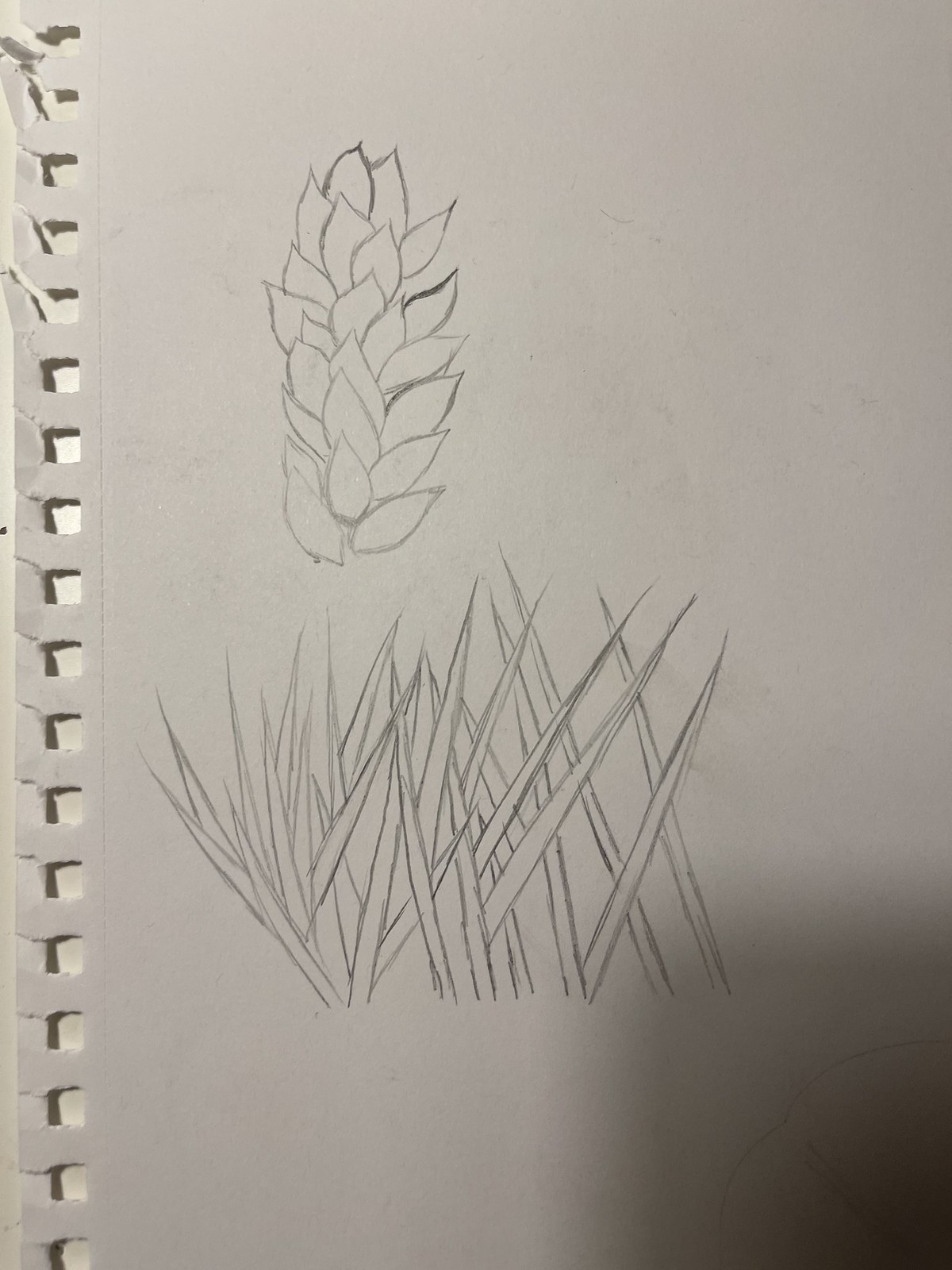This photographic image showcases a page torn from a spiral notebook, with a slightly ragged perforated edge indicating it could have been detached more neatly. The white page features a detailed pencil drawing, with distinct shadows cast on it from the camera. At the bottom of the page, delicately crafted blades of grass are depicted. Central to the drawing is a flower-like plant with long, slender leaves extending upwards along its sides, culminating in a shape reminiscent of a pine cone or a cone. Erase marks and light shadowing add texture and depth to the entirely pencil-rendered artwork.